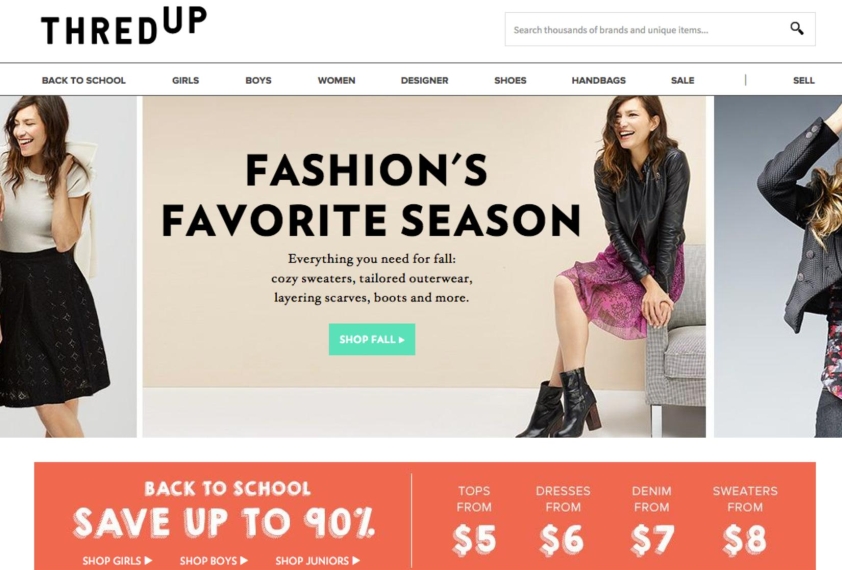The image appears to be a screenshot of an online store's webpage, specifically from ThredUp, which is indicated by the logo at the upper left corner. To the right of the logo, there is a search bar with a magnifying glass icon positioned at the left end. Below the search bar, there is a navigational menu with clickable options in black text for categories such as "Back to School," "Girls," "Boys," "Women," "Designer," "Shoes," "Handbags," "Sale," and "Sell."

The main content area features three photographs. The first image on the left is a vertical, narrow rectangle showing a woman with long brown hair, wearing a light-colored short-sleeve shirt and a dark skirt. She is smiling, looking to the left, and her pose has her legs crossed and one hand toward her hair.

The central image is a larger, horizontal rectangle with a tan background. It is captioned "Fashion's Favorite Season." This photo features the same woman sitting on the edge of a gray chair to the right side of the frame. She is dressed in a pink skirt, a long black shirt or jacket, and shiny black knee-high boots. Her arms and legs are crossed, and she is smiling while looking to the left. Below the main title, there is a brief description and a green button labeled "Shop Fall," inviting users to click and browse the fall collection.

The image on the far right is a partial view, revealing only part of the woman's black jacket, her arm, and some hair, against a gray background. Her face is not visible.

At the bottom of the screen, a large orange banner with white text announces back-to-school savings of up to 90%, highlighting deals such as tops starting at $5, dresses at $6, denim at $7, and sweaters at $8. The banner also includes buttons for "Shop Girls," "Shop Boys," and "Shop Juniors."